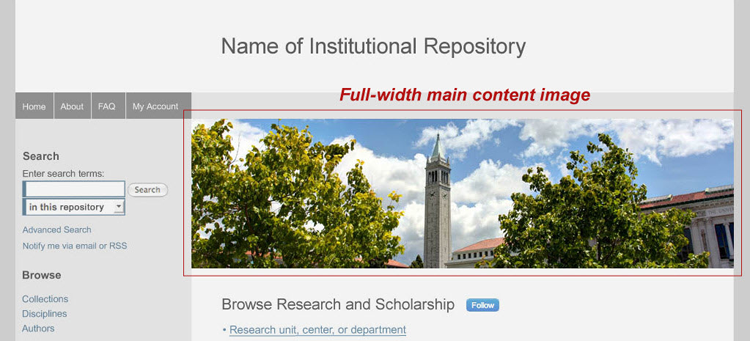The screenshot is from a website, displayed in full color, with a variety of gray tones forming the background. The website header features a light gray section across the top, where centrally placed black text announces "Name of Institutional Repository." Along the left side, a medium to dark gray sidebar houses navigation tabs with white text, reading: "Home," "About," "FAQ," and "My Account." 

Further down this sidebar, a slightly lighter gray background supports additional search functionalities. This area includes prompts with the black text "Search" and "Enter search terms," accompanied by a search box. Below this, blue text offers options for "Advanced Search" and notifications: "Notify me via email or RSS." Continuing with the navigation, black text labels a section "Browse," under which blue links list "Collections," "Disciplines," and "Authors."

Adjacent to the left sidebar, a prominent image captures the roof of a large building, flanked by two trees beneath a blue sky spotted with clouds. Above the image, red text boldly states "Full Width Main Content Image." Below this image, black text invites users to "Browse Research and Scholarship," followed by a blue button labeled "Follow." Completing the setup, blue text directs users to "Research Unit, Center, or Department."